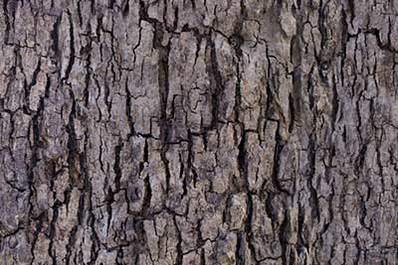This close-up photograph captures the intricate details of a tree trunk's bark, filling the entire frame with a textured tapestry of nature. Taken in bright daylight, the image reveals a complex interplay of deeply etched grooves, cracks, and geometric shapes, accentuating the bark's rugged surface. Various shades of brown, gray, and hints of ashen tones blend naturally, creating a multi-dimensional effect. The bark appears worn and weathered, resembling dried-out clay or baked dirt, with numerous vertical and horizontal lines forming a mosaic-like pattern. The image includes areas of smooth bark interspersed with rough, protruding sections and a mix of small and large cracks. A round hole is visible, adding to the bark's character. The photo focuses solely on the tree trunk, emphasizing its aged, natural beauty without any background distractions.